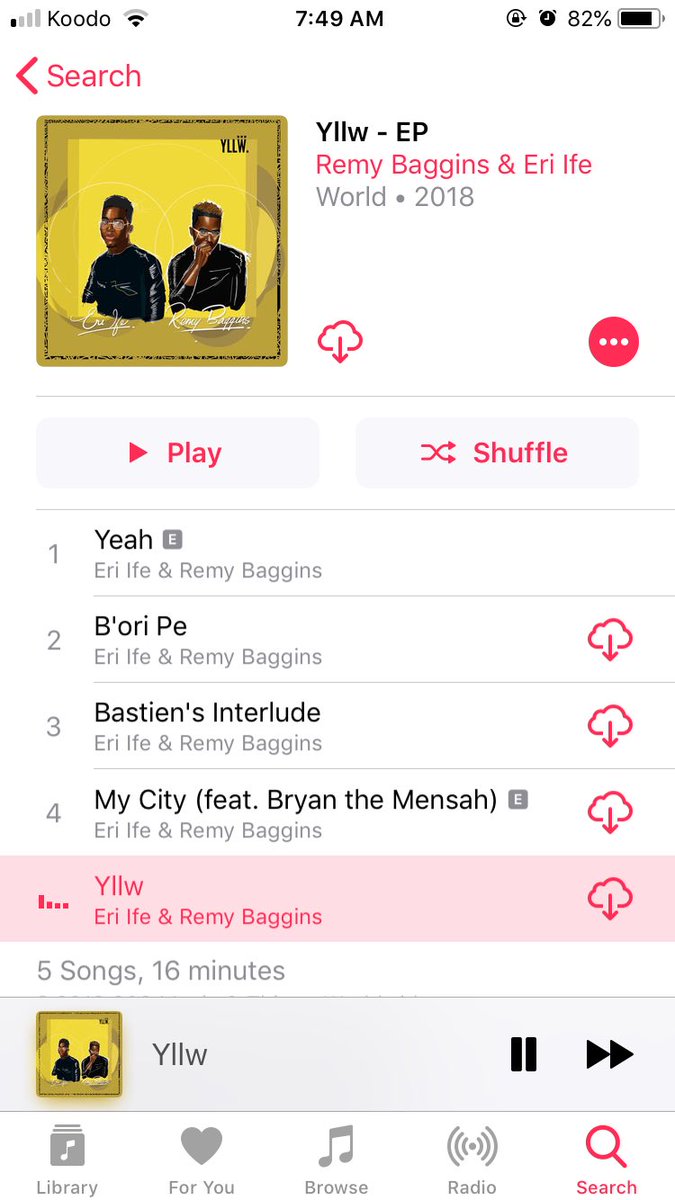This screenshot captures a smartphone display at 7:49 AM with an 82% battery level, serviced by Kudo, and currently running a music application. The app interface features a prominent search function on the top left, allowing users to navigate back to their main music library. 

The central focus of the screen is the album "Yelloo EP" by Remy Baggins and Ari Ife, released in 2018. The album cover is strikingly golden, featuring the two artists dressed in black, posing confidently inside a golden frame. 

At the bottom of the screen, a list of tracks from the album is shown, with the currently playing track titled "Yelloo". Other tracks available in the album are "Yeah," "Bori," "P," "Bastions," "Interlude," and "My City".